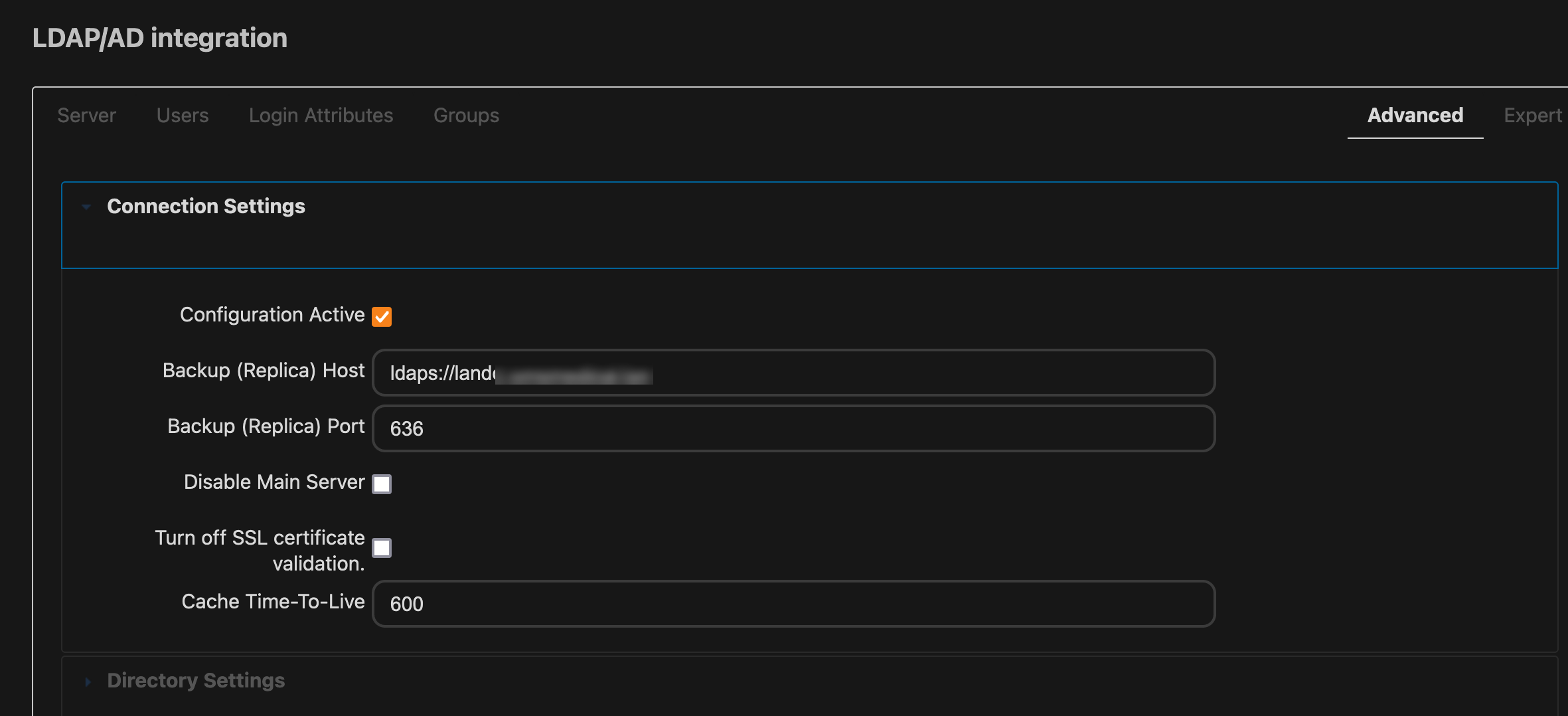**Descriptive Caption:**

The screenshot showcases a user interface intended for LDAP/AD integration configuration, displaying a clean and organized layout on a black background with white text. In the upper left-hand corner, the title "LDAP \ AD Integration" is prominently displayed in white lettering. Beneath the title, a white line outlines a square and under it, navigation tabs are listed: "Server," "Users," "Login Attributes," "Groups," with "Advanced" in bold and "Expert" next to it on the far right. Below the "Advanced" tab, another white line appears.

A long blue rectangle underneath features the text "Connection Settings" in bold white. Below this, the configuration status is marked as "Configuration Active," indicated by an orange square with a white checkmark.

Following this, the term "Backup (Replica)" appears above fields for "Host," in which a long white rectangle displays an incomplete, blurred-out URL starting with "IDAPS://\L" among other escaped backslashes. Below it, the "Backup Replica Port" is specified, showing "636" in another white rectangle.

The interface further includes options such as "Disable Main Server," and "Turn off SSL Certificate Validation," each accompanied by an unselected white square. Finally, the section "Cache Time to Live" shows a value of "600" in a long white rectangle, with "Directory Settings" labeled underneath it.